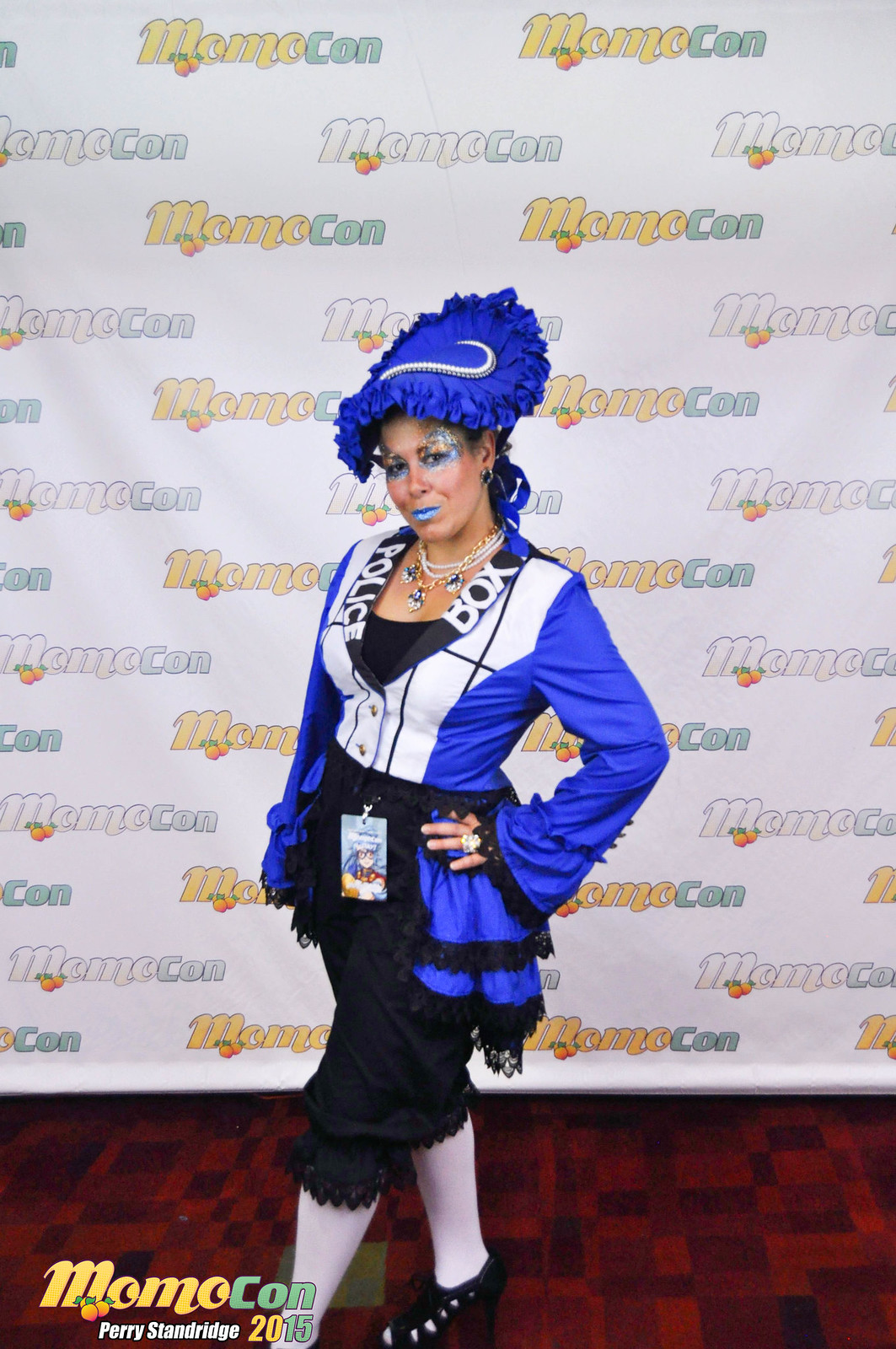A Caucasian woman in her 40s, likely a cosplayer, stands poised on a red carpet in front of a tall white banner adorned with the "Momocon" insignia and images of oranges, alongside the text "Momo Khan, Perry Standridge, 2015" in yellow, blue, and white letters at the bottom left. Her left hand rests confidently on her hip, her left foot forward, and her right foot tucked back. She dons an intricate outfit featuring black capri pants with lace trimming, black high heels, and white stockings. Her attire includes a distinctive blue and white top with "Police Box" emblazoned on the collar, indicating a possible "Doctor Who" reference, accompanied by a black undershirt. Her accessories comprise a white necklace with three dangling blue elements, possibly badges or tags, and a sizable ring on her hand. Completing her look is a blue vintage hat, blue lipstick, sparking eye makeup, and a clip on her waistband, possibly a badge or decorative element. The backdrop and the woman's elaborate outfit suggest she is attending an anime convention or similar event, embodying a character with a blend of whimsical and chic elements.